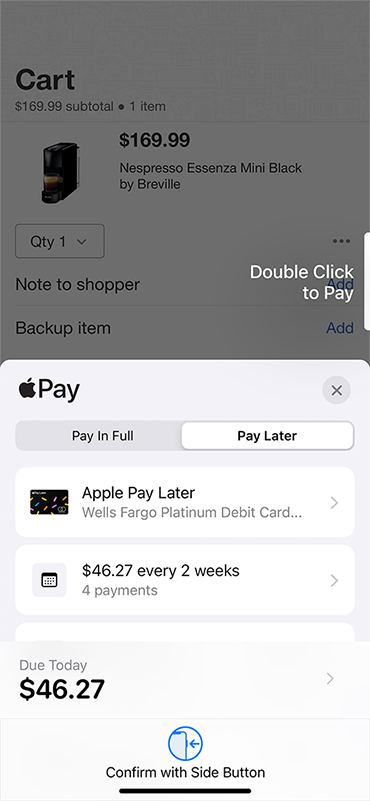This screenshot showcases an e-commerce checkout page with a gray background on the top half and a light gray background on the bottom half. 

At the top, approximately eight lines down on the left side, bold black large letters read "CART." Directly beneath it, in smaller black text, is the subtotal displayed as "$169.99." To the right of this, a black circle indicates the quantity of items.

Below, the featured item is a Nespresso coffee maker displayed as an image. To its right, in large bold black text, the price is listed as "$169.99." Further details describe the item as "Nespresso Essenza Mini Black by Breville."

Directly underneath, a drop-down box is available, outlined in gray, showing "QTY 1" with a down arrow for selection. Below this, in black text, the options "Note to shopper" and "Backup item" are available, both adjacent to a blue "Add" button. On the "Note to shopper" line, there is a white "double click to pay" wording above the blue "Add" button.

On the bottom half, located in the left-hand corner, is the Apple logo followed by bold black text reading "Pay." Two payment buttons are positioned side by side: the left button with a gray background, saying "Pay in Full," and the right button with a white background, saying "Pay Later."

Below these buttons, there are two visible rectangles, with the top of a third one slightly showing. The first rectangle features an icon to the left with a colorful design, and next to it, the bolded black text "Apple Pay Later." Underneath, in gray, it reads "Wells Fargo Platinum Debit Card..." with a right pointing arrow at the end of the line.

The second rectangle includes an image of a square resembling a calendar. To the right, the bold text displays "$46.27 every two weeks," followed by "For 4 payments" in gray and another right pointing arrow.

At the bottom of the screen, a gray background contains the text "Due today," followed by the bold black amount "$46.27."

This detailed caption elucidates all visual and textual elements present in the screenshot, ensuring comprehensive understanding.